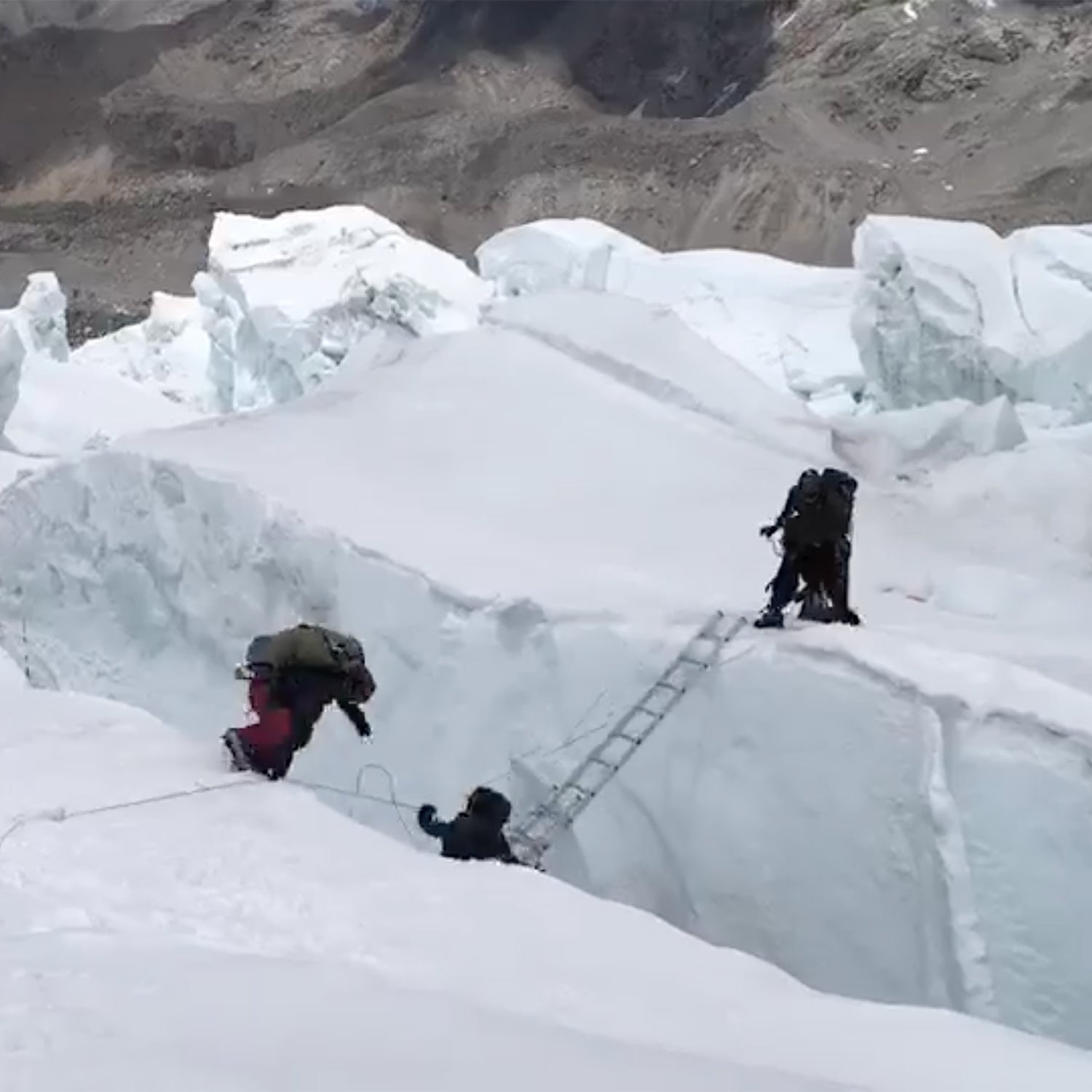In this photograph set in a high-elevation, snowy mountain environment, three individuals are attempting to traverse a steep gorge using a makeshift bridge constructed out of a ladder. The bridge spans a deep crevice, which separates two snowy sections of the mountain. The climbers are equipped with heavy-duty hiking gear and protective clothing, indicating their serious commitment to the arduous snow trek. The scene showcases a stark contrast between the white snow blanketing the bottom part of the image and the gray, rocky cliff face in the background. Two of the climbers are positioned on one side of the gorge, while the third is on the opposite side, each engaged in carefully navigating or supporting each other as they progress. The image captures a moment of intense focus and teamwork amid the challenging mountainous terrain.